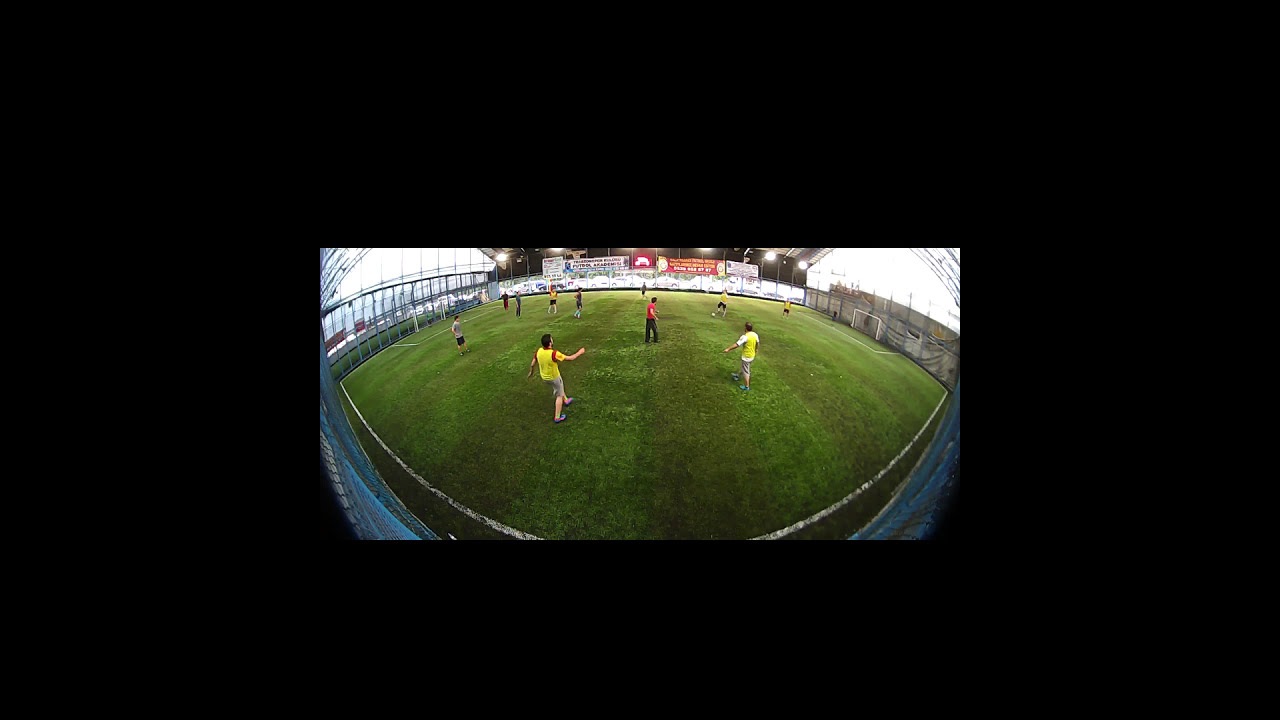The photograph, likely taken from a security camera with a fisheye or wide-angle lens, captures a detailed, slightly distorted image of a soccer game, creating a curved appearance around the edges. The setting appears to be an indoor soccer field, characterized by its alternating dark and light green striped astroturf and white painted lines. The scene is bustling with activity: players in yellow shirts and shorts engage in the match, alongside an individual in black pants and a red shirt, potentially a referee or coach. The soccer goals are positioned to the left and right, and the field is enclosed by tall fencing. In the background, blurred signage in white and red, possibly advertisements or sponsorship, can be seen amidst stands or spectator seating. The atmosphere is overcast with cloudiness, suggesting artificial lighting is used to illuminate the field, enhancing the visibility of the ongoing game.